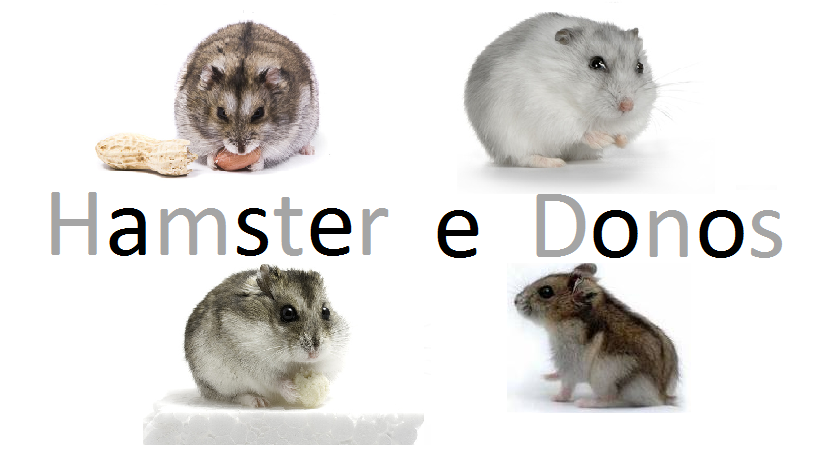The picture features four adorable hamsters arranged in a square layout against a white background, with writing in the center of the image. The text, "Hamster A Donos," is displayed in alternating gray and black letters, with the letters A, S, E, E, and O in black while the others are in gray. The hamsters are divided by this text, with two on the top row and two on the bottom. 

The top left hamster, brown with a white underbelly, is seen nibbling on a peanut, with the shell visibly to its left. The top right hamster, mainly white with some gray fur and dark eyes, is adorably looking to the right with its tiny claws raised as if begging. 

In the bottom row, the left hamster, a bit grayer in fur compared to the top right hamster, appears to be sitting on a towel or cushion. The last hamster on the bottom right is mostly brown with a white underbelly and is looking off to the left side. Each hamster has distinct features, such as their furry coats, little ears, and irresistibly cute faces.